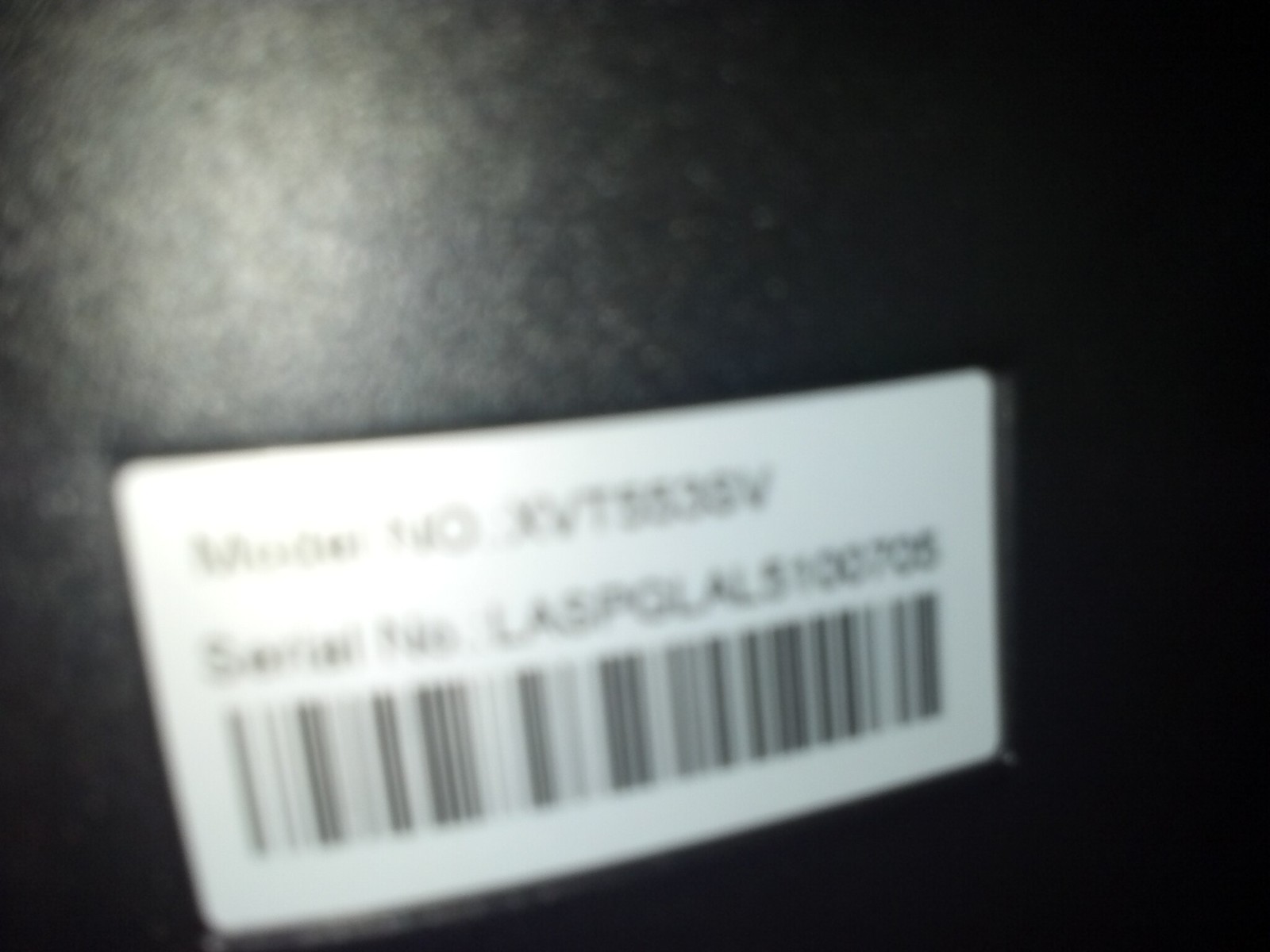This image appears to be an out-of-focus shot of the back of an electronic device, set against a shiny black backdrop. The glossy surface of the backdrop is reflecting the camera flash, adding to the overall blur of the image. There is a rectangular, horizontal white label with black text on the device, though the exact details are indistinct due to the lack of focus. The label seems to contain the phrases "Model No." and "Serial No.," presumably identifying the model number and serial number of the device. Despite the fuzziness, these elements suggest the item could be the rear panel of a computer or a similar electronic appliance.